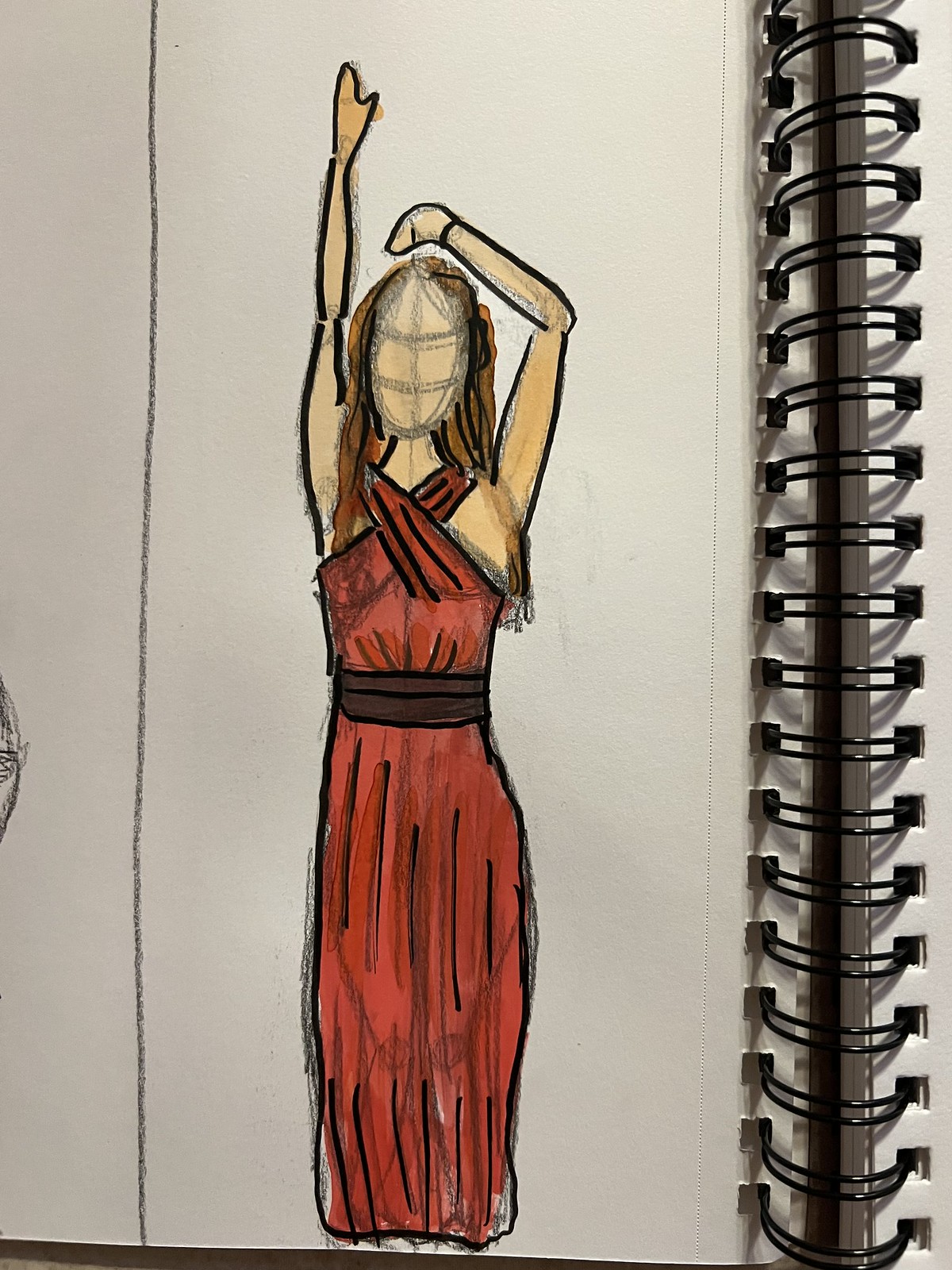This image features a hand-drawn fashion illustration in a spiral-bound sketchbook. The sketch, likely by a young teenager, showcases a woman in a red crisscross halter top dress. The dress features a bodice with material crossing over the breasts, fastening at the back, and a partially sheer skirt that hints at the figure's knees and legs beneath. A dark brown or black sash accentuates the waist. The woman is depicted with her right arm extended straight up and her left arm bent at the elbow, resting near her ear, giving the impression of a dynamic pose. Her hair is brown, though her face remains unfinished with only proportional guidelines sketched in. The drawing is part of a larger sketchbook, occupying one portion of a page divided by a pencil line, with the iconic spiral binding visible on the right-hand side.